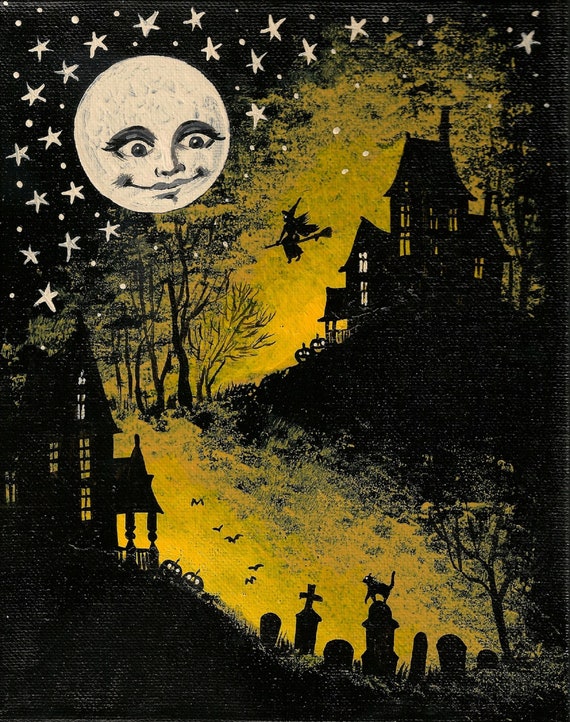The image is an artistic Halloween illustration set against a black nighttime background, centered around a white moon with a smiling, detailed face in the upper left-hand corner. The moon, drawn with large eyes, a nose, and a semi-smiling mouth, is surrounded by childlike, sparkling stars. Prominently featured in the middle is a yellowish silhouette scene: a witch flying on a broomstick near a Victorian-style house perched atop a hill, surrounded by bare trees and pumpkins. Below, at the bottom of the hill, another house stands near a graveyard with a cat perched on one of the tombstones. Bats can be seen flying in the sky, adding to the eerie atmosphere.